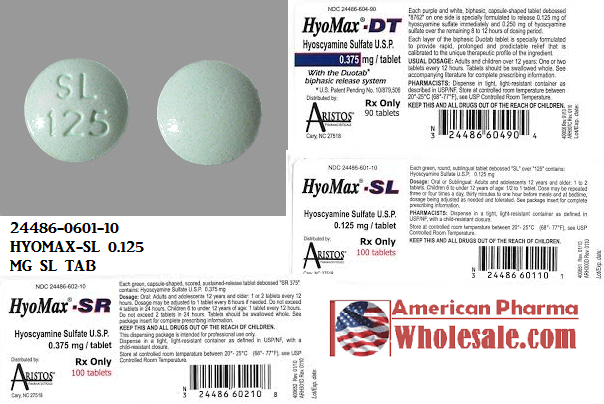The image features a detailed label of a medicinal product with the following information:

- **Top Left:** A gray and green emblem labeled "SL 125".
- **Center:** A label for "Max-Sign," presented in blue text with the identifier "244860 - 601-10".
- **Main Section:** The description "Hi-O Max-SL 0.125 mg," followed by "SL Tab." Adjacent to this, it reads "2445 Hi Max-SR Hi-O 6".
- **Specific Details:** "Hi-O Max-SR, Sulfate USP, 0.375 milligrams per tablet, RX Only, 100 tablets," developed by Aristos Pharmaceuticals.
- A note mentions "Each capsule is a scored, sustained-release tablet." The dosage instructions for adults are "1 to 2 tablets every 12 hours. Dosage may be adjusted to 1 tablet every 8 hours if needed. Do not exceed 4 tablets within a 24-hour period. Not for pediatric use."
- **Bottom Right:** Identifies "Hi Max-DT" and "Hi Max-SL." In red text, it reads "American Pharma Wholesale."
- The label also shows an American symbol, highlighting the origin of the pharmaceutical distributor.

The label is laden with technical and dosage information, suggesting this is a prescription-only medication designed for adult usage, with strict dosage guidelines provided.